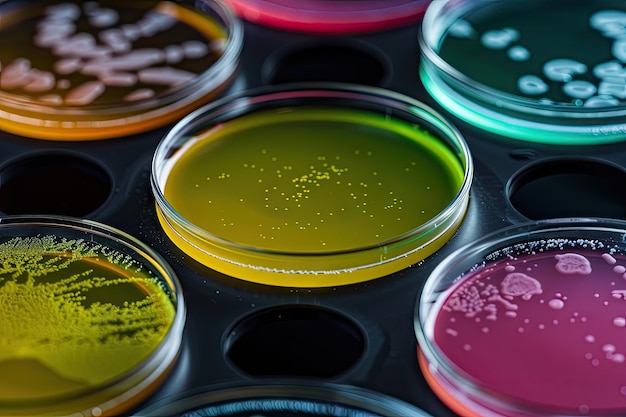This photo showcases an up-close view of five petri dishes neatly arranged in a black metal or plastic container, resembling the five dots on a die. Each petri dish contains a different colored substrate: a pink dish in the bottom right, a teal or cyan dish in the top right, an orange dish in the top left, and two yellow dishes, one in the center and one at the bottom left. The yellow dish in the center has smaller white specks indicating some culture growth, while the yellow dish in the bottom left exhibits a dense, full-grown bacterial colony. The teal dish on the top right displays larger circles of microbial growth, and the orange dish in the top left has more significant white specks growing together. The pink dish at the bottom right shows a comparatively higher amount of white microbial growth, about three to four times more than the yellow dish in the center. The container ensures these petri dishes are evenly spaced and securely held.